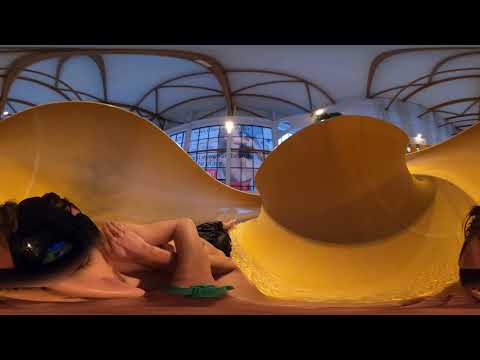The image appears heavily distorted, likely due to the lens used, leading to a surreal composition. In the background, a white ceiling with brown beams forms a multifaceted pattern, accompanied by windows that frame an advert of a female model. Dominating the foreground, a person is seen with their legs and arms crossed and folded, adding to the sense of disarray. To the right, an enigmatic element that resembles a yellow, round shape with spoon-like extensions at either end, further adds to the visual confusion. Below this shape, more yellow coloring blurs the details. On the left side, another black circular form is visible. Distorted black bars frame the top and bottom of the image, emphasizing its 16x9 landscape orientation. Overall, the image's chaotic elements and distortion make it challenging to decipher.